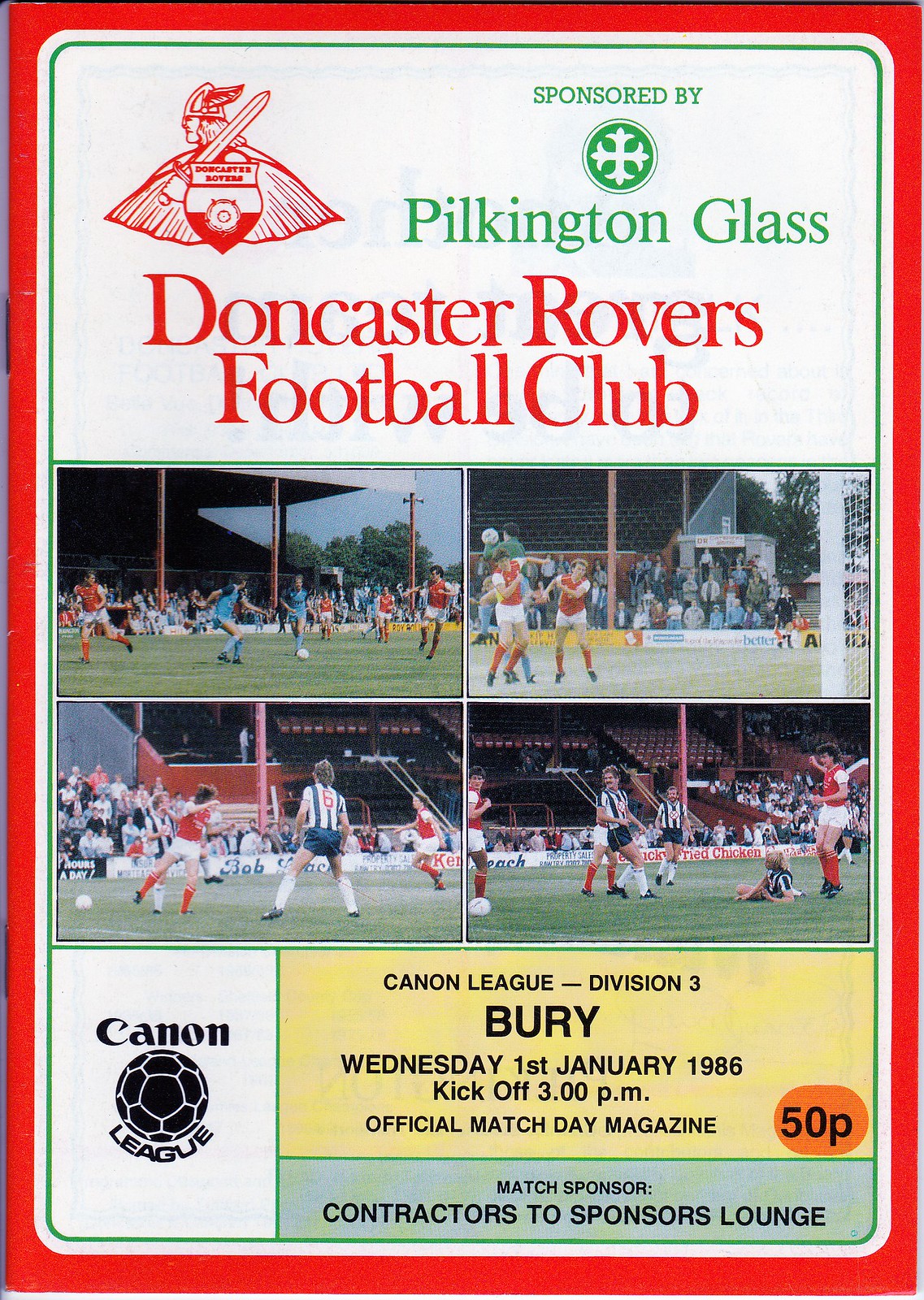This is the cover of an official match day magazine for a soccer game featuring the Doncaster Rovers Football Club. The cover has a red border and a white text area at the top, prominently displaying the club's logo, which depicts a Viking holding a sword in front of a shield. To the right, green text announces "Sponsored by Pilkington Glass," accompanied by their logo—a green circle enclosing a Celtic cross-like design. Below this, "Doncaster Rovers Football Club" is printed in bold red text.

In the central section, four photographs depict various soccer matches, showing players in red jerseys of the Doncaster Rovers competing against teams in blue and striped jerseys. The images capture dynamic moments from the soccer field, illustrating different players and game situations.

The bottom of the cover is organized into distinct advertising sections. A yellow text box lists event details, reading: "Cannon League Division III, Bury, Wednesday 1st January 1986, kickoff at 3 p.m., official Match Day magazine, 50 pence." To the left of this, the Cannon League logo features the word "Cannon" above an illustration of a soccer ball, with "League" written below. Finally, a green text box at the very bottom states: "Match Sponsored Contractors to Sponsor Lounge."